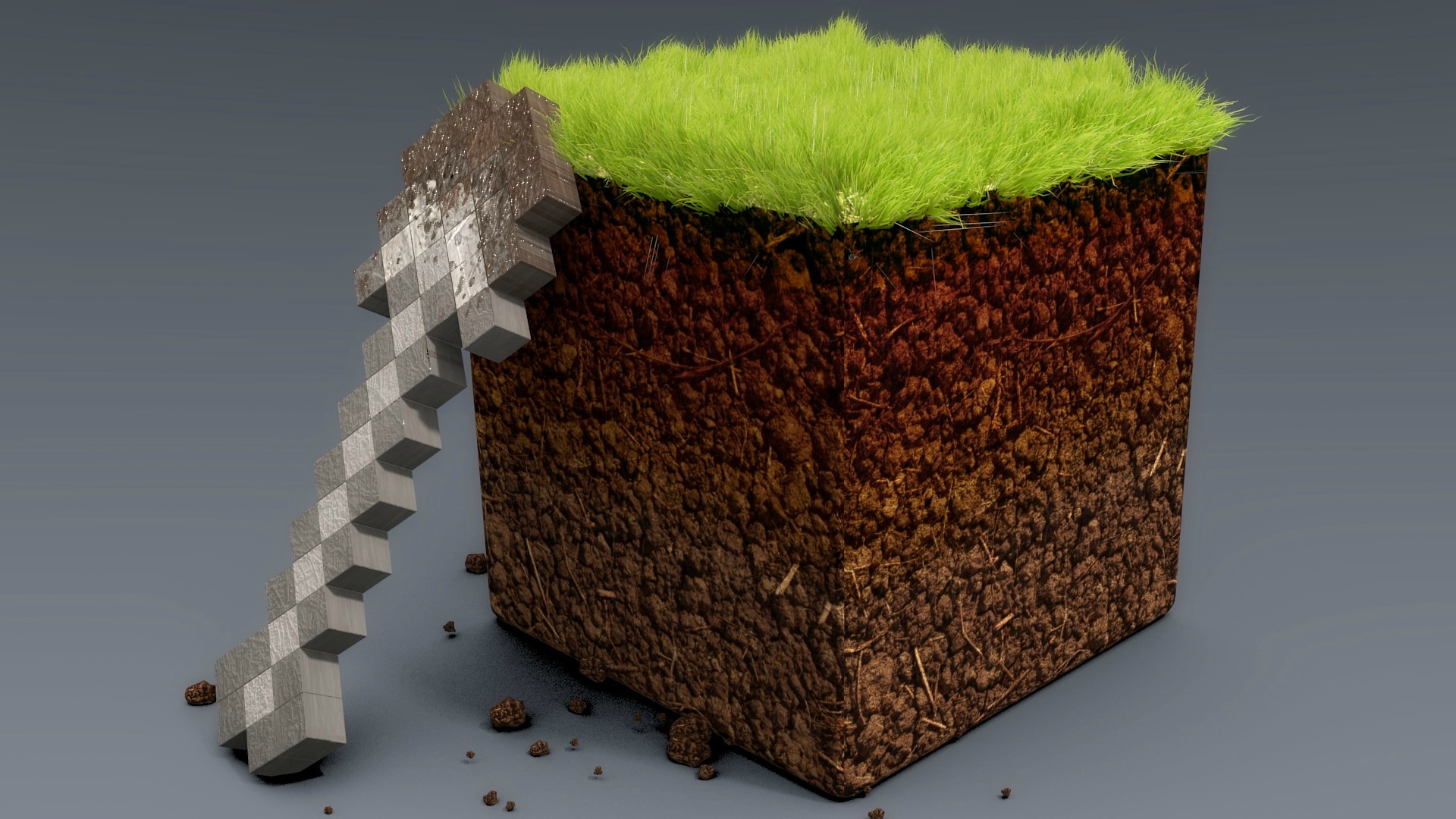A captivating and surreal composition features two computer-generated images set against a serene medium slate blue backdrop. The primary image showcases an artificial cube of earth with distinct layers of texture — its base is a light to medium brown, depicting dry soil, transitioning into a slightly darker, moist layer above. This nuanced gradation suggests recent watering. Atop the cube, a luxuriant growth of thick, light green grass flourishes, balancing the earthy tones below. The scene is enhanced with fragments of the brown soil scattered on the surface where the cube rests.

Adjacent to the earthy cube, an intriguing construction of imaginary blocks leans against its side. These blocks are a mix of medium and light gray, mimicking masonry. The structure begins with a three-block wide base and ascends into a tower, narrowing to two blocks across, ultimately merging with the cube's earthy summit. The juncture where the tower meets the cube is adorned with additional soil, blurring the lines between the distinct elements and adding to the composite's enigmatic charm.